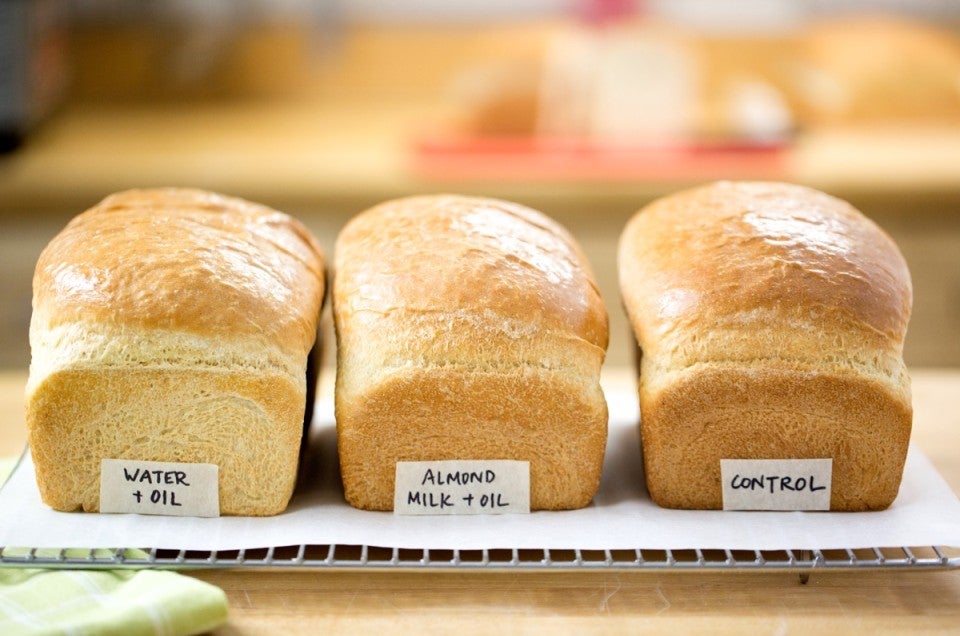This photograph portrays three freshly baked loaves of bread, presented in a close-up view. Each loaf rests on white parchment paper atop a silver metal cooling rack, which itself is set on a light brown wooden table covered partially by an olive green cloth. The loaves, golden brown with darker corners, exude a shiny, basted top. Rectangular labels are placed in front of each loaf, written in black ink: the left reads "water plus oil," the middle reads "almond milk plus oil," and the right reads "control." The setup is illuminated by bright lighting, suggesting a kitchen or bakery setting. The background is blurred, revealing a hint of another table and indistinct objects, possibly indicating a bustling kitchen environment.